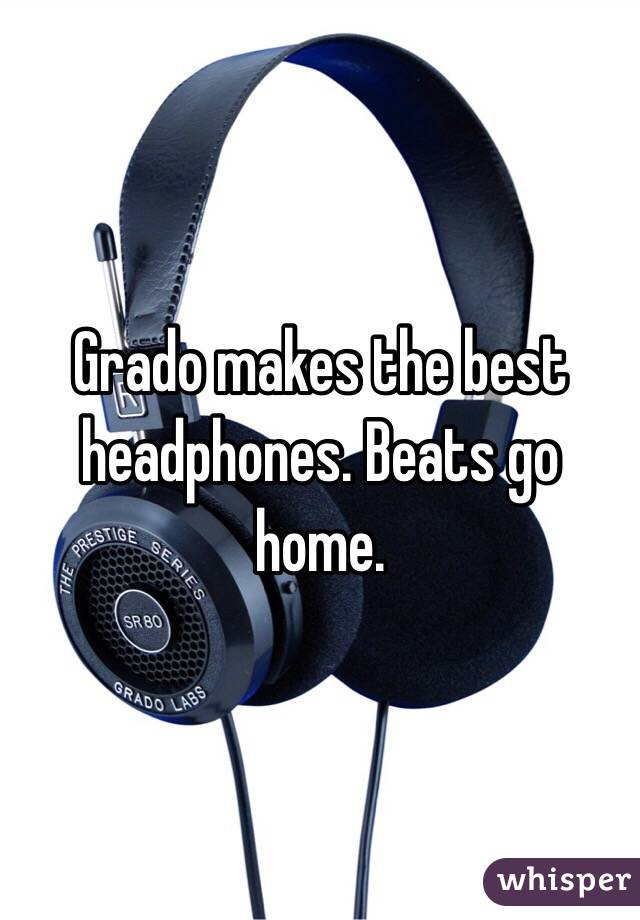This image is an advertisement for Grado headphones, prominently featuring a pair of black, over-ear headphones against a dark background. The headphones have a leather strap running across the top and circular ear cups. The right ear cup displays the text "The Prestige Series, Grado Labs, SR-80" in white. The textured section of the ear cup adds a tactile design element to the headphones. Angled slightly toward the viewer, the headphones also include a feature resembling an antenna, possibly a microphone. Across the middle of the image, bold white text with a black outline declares, "Grado makes the best headphones. Beats go home," emphasizing Grado's quality over the well-known Beats brand. In the bottom-right corner, there's a logo encased in a purple box with the word "Whisper" in lowercase white font.